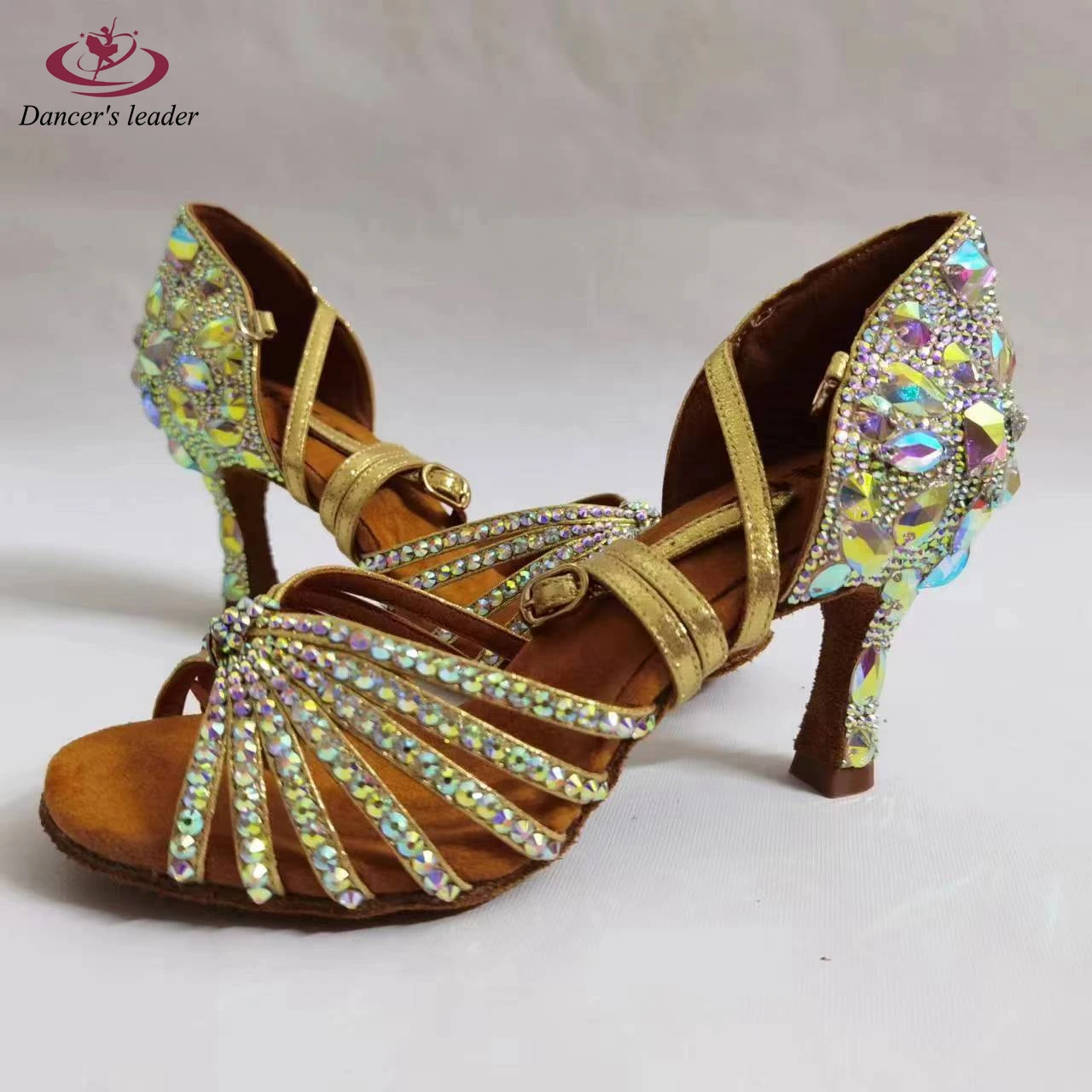The image is an advertisement featuring a pair of vintage high heel shoes positioned centrally. In the upper left corner, there's a logo with the text "Dancer's Leader." Dominating the scene are two high heels, prominently adorned with glittering rhinestones and faux gemstones of various colors such as clear, yellowish-blue, and purple. The shoes feature intricate leather straps embedded with shimmering glitters and tiny diamonds. The nearest shoe presents a detailed side view, showcasing its sparkling embellishments from the toe to the heel, while the second shoe appears slightly behind to the left, partially obscured but similarly decorated. Both shoes cast shadows, enhancing the realistic yet possibly computer-generated aesthetics of this visually striking and nostalgic advertisement.